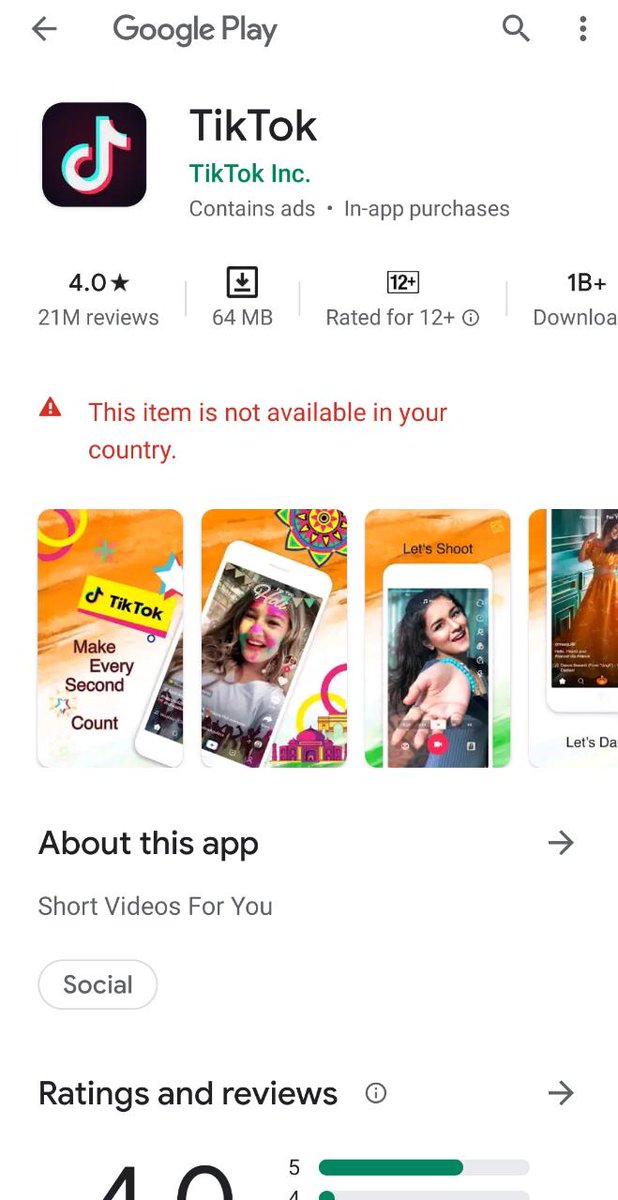The image depicts a screenshot of the Google Play Store page for TikTok. The page prominently features the TikTok logo and states that the app "contains ads" and offers "in-app purchases." The app has a four-star rating based on 21 million reviews and requires a 64-megabyte download. A caution triangle icon with a message indicates that "This item is not available in your country." The page showcases several promotional images of the app, mostly featuring young women dancing and enjoying themselves. There's an "About this app" section that users can click for more information, and a "Social" tag categorizing the app. The bottom portion of the page shows a snapshot of the app ratings, with a noticeable spread of five-star and four-star reviews, indicating a mix of user feedback. The context suggests that the user attempting the installation is in a region where TikTok is either banned or restricted.